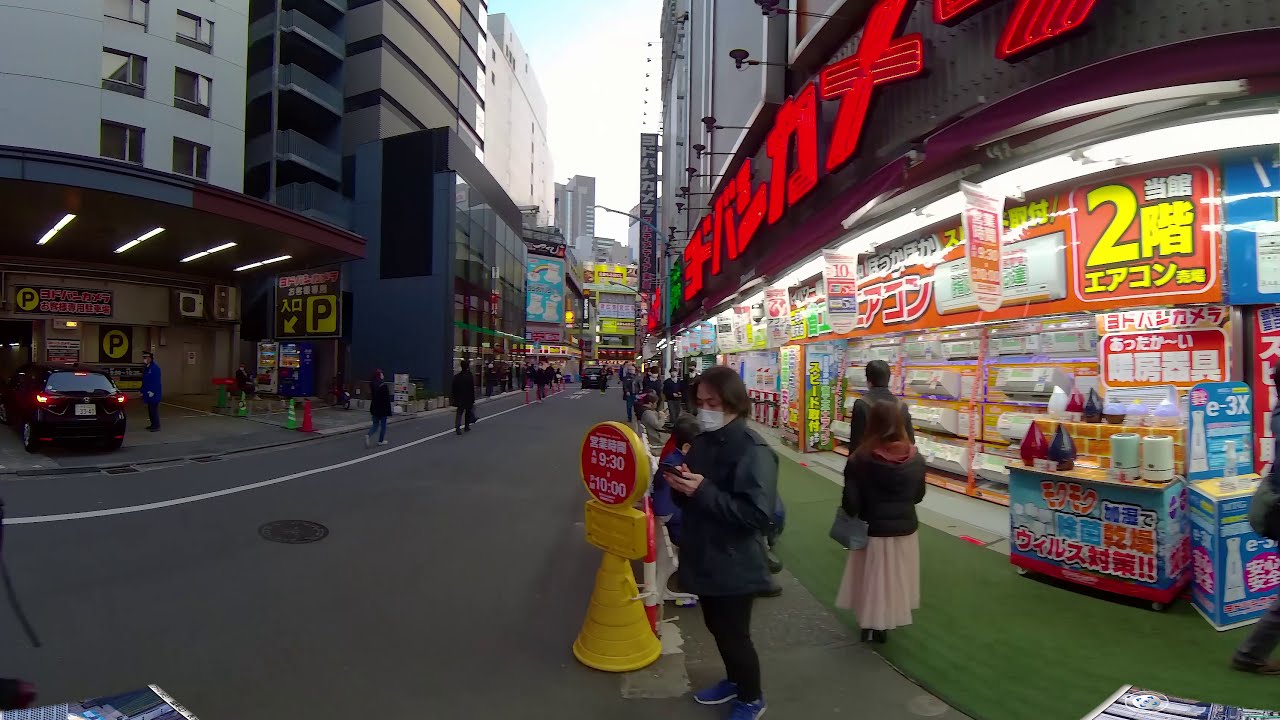The image captures a bustling street scene in Japan, with a vibrant and densely packed city setting. On both sides of the one-lane street, various storefronts and stalls are adorned with numerous advertisements and Japanese signage, creating an atmosphere of commercial overload. A yellow sign with a red circular top displaying the numbers "9-30" and "10-00" adds to the street's character. 

Buildings rise on both sides, indicating the urban nature of the scene. On the left side, there is a parking garage where a car is entering, guided by a man possibly directing the vehicle into the space. Above the entrance, a sign with a "P" likely designates the parking area. Nearby, vending machines in blue and white provide additional details of daily life.

In the foreground, a woman dressed in a white skirt, black jacket with a brown hoodie underneath, is preoccupied with her phone while carrying a purse. Along the green walkway on the right, more people, dressed for cooler weather, are seen walking and carrying bags. One man, also on his phone and wearing a mask, adds to the scene's contemporary feel. The stores on the right include one selling air conditioners, adding to the variety of the marketplace. The backdrop consists of more buildings and banners, completing this vivid portrayal of a Japanese city street.